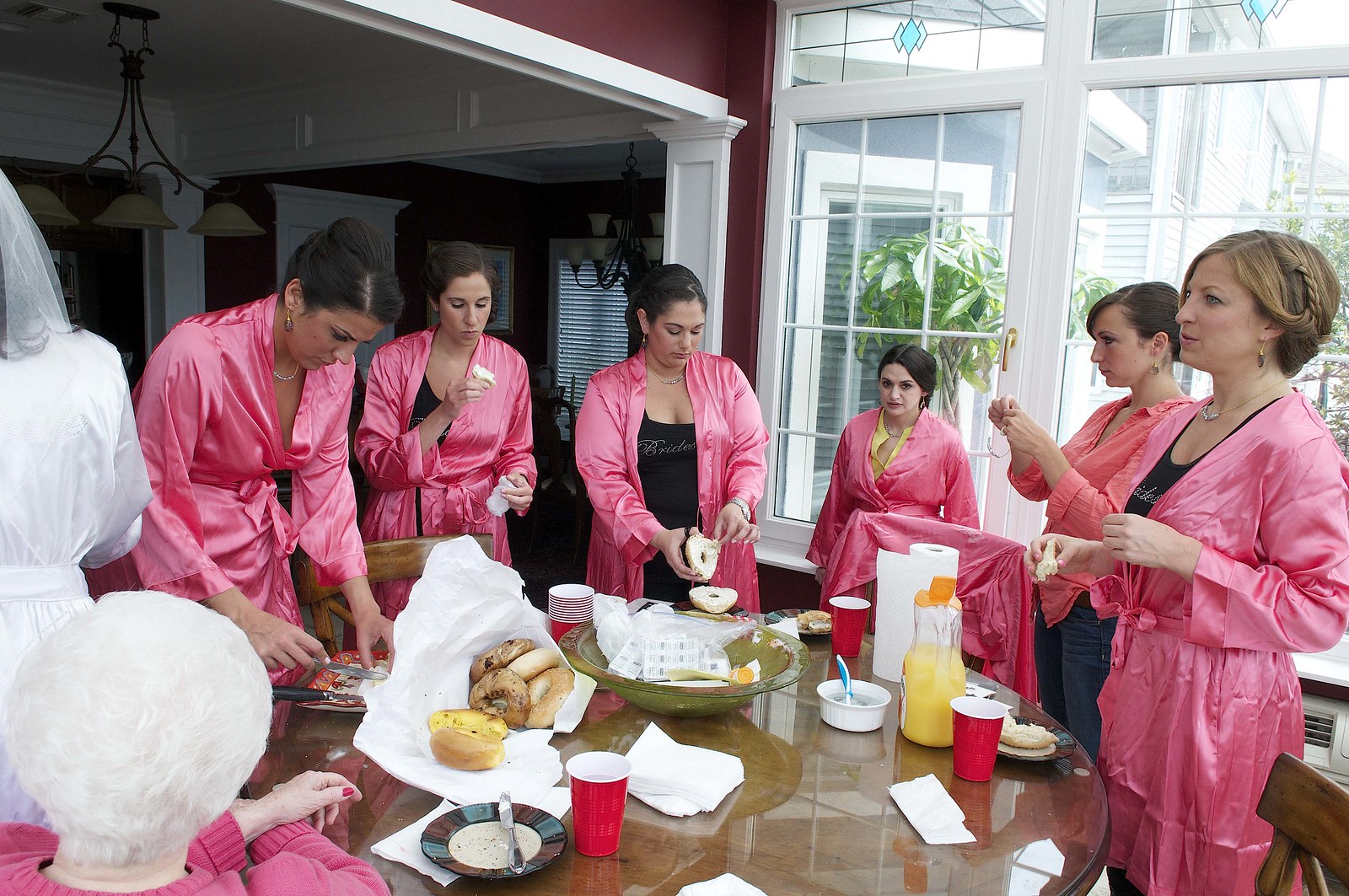In this photograph, six women, each wearing identical silky pink robes with tied sashes, stand around a wooden dining room table laden with an assortment of morning-style food and party supplies. Some of the women are fully dressed underneath their robes, while others appear to be in pajamas or lingerie. They all have dark hair, either short or pulled back. The table is covered with various bowls, plates, bottles, and cups, including stacks of red plastic party cups with white interiors. Centrally placed is a bowl filled with small packets, likely containing salt and pepper, as well as a napkin holding a large loaf of bread and a small brioche bun. On the right side of the image, a large two-panel window divided by white wood into smaller sections reveals a green bush and a portion of the front yard outside. On the left side, a darker painted wall with white wooden trim features an archway leading into a larger room. The scene suggests a relaxed gathering, possibly a bridal party preparing for a spa day or retreat, evidenced by the identical robes and the festive table setting.